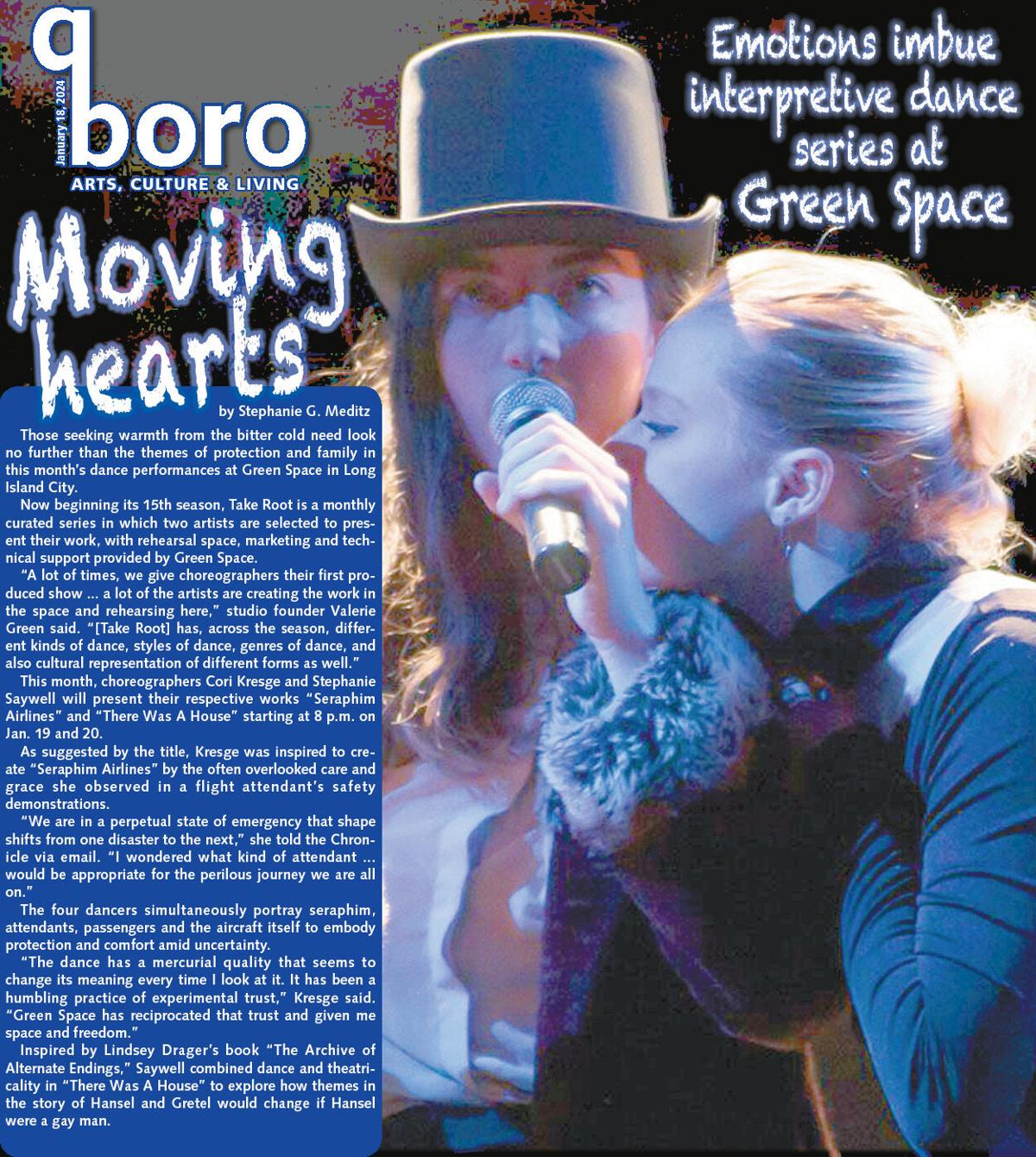The magazine cover for BORO showcases Kuboro Arts, Culture, and Living, with an emphasis on the Moving Hearts and Emotions Imbue Interpretive Dance Series held at Green Space in Long Island City. The upper left corner features the title "BORO" against a gray background with "Arts, Culture, and Living" beneath it in small blue letters. The right corner prominently highlights, in white letters on a black background, "Emotions Imbue Interpretive Dance Series at Green Space." 

Central to the cover is a striking image of a man and a woman. The man, wearing a gray top hat and a purple or burgundy coat with blue sleeves and fur fringe around the ankles, holds a microphone to his mouth with his left hand. The blonde-haired woman rests her hand on his bicep and leans into the microphone. She is adorned in a blue shirt with a white circle around the neckline and has her hair pulled back in a bun.

The left column under "BORO" in white letters continues with "Moving Hearts," and the first paragraph teases the article, stating: "Those seeking warmth from the bitter cold need look no further than the themes of protection and family in this month's dance performance at Green Space in Long Island City." The magazine proceeds to detail the dance series "Take Root," now in its 15th season, which provides selected artists with rehearsal space, marketing, and technical support from Green Space. 

A featured article by Stephanie C. Meditz further explores the series, shedding light on the current performance by choreographers Corey Kressig and Stephanie Saywell, respectively presenting "Seraphim Airlines" and "There Was a House." Kressig’s piece, inspired by the vigilance of flight attendants, examines the transient emergency states of life, while Saywell reinterprets the narrative of Hansel and Gretel through a contemporary lens, inspired by Lindsay Dagger's book. Quotes from the artists and series founder Valerie Green emphasize the varied and culturally rich nature of the performances.